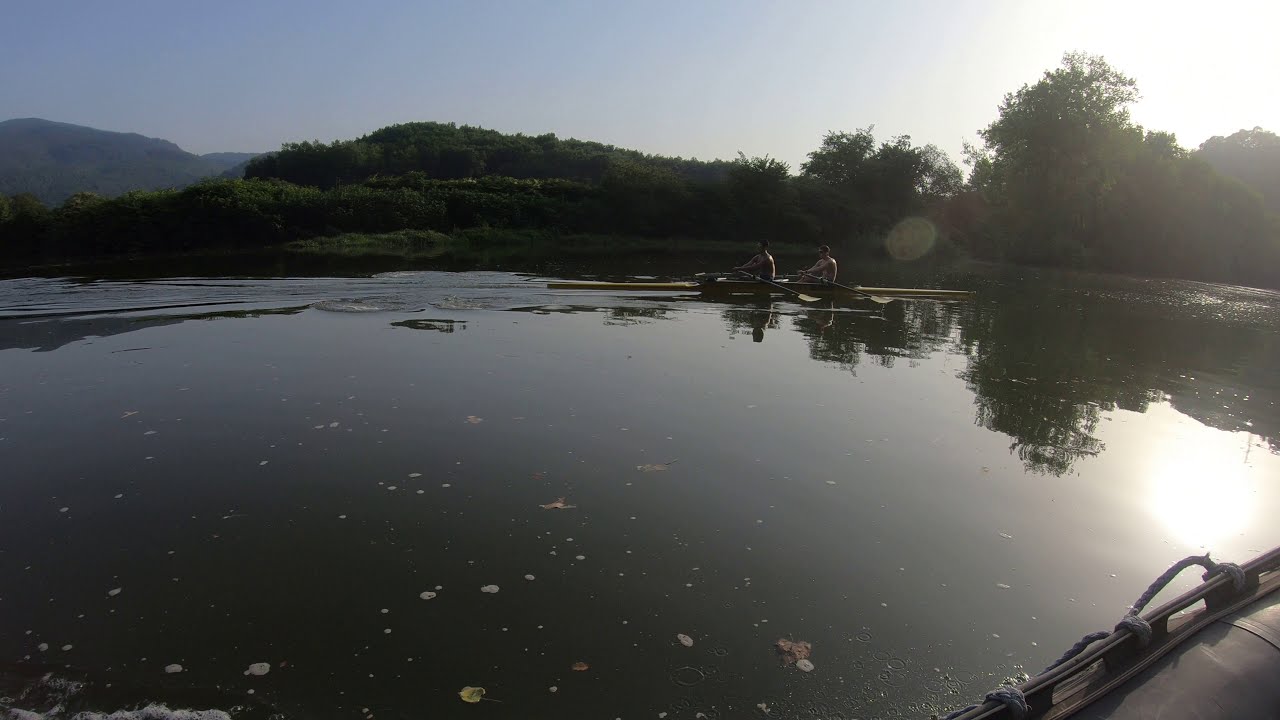The image captures a serene lake scene with dark, murky green water dotted with white suds and bubbles. In the foreground, the photo appears to be taken from a kayak, as suggested by the outline in the bottom right-hand corner. Two people in a kayak, both shirtless, paddle toward the left-hand side of the image. The water is calm and strewn with leaves. The setting sun, visible in the upper right-hand corner, casts a soft reflection on the lake’s surface, adding a touch of warmth to the otherwise cool-toned palette of grays, greens, and blues. In the background, there are outlines of hills and trees to the right, with a larger hill or mountain visible in the upper left. The upper half of the image features a mostly clear blue sky, with a slight whiteness surrounding the sun, creating a tranquil, late afternoon atmosphere.